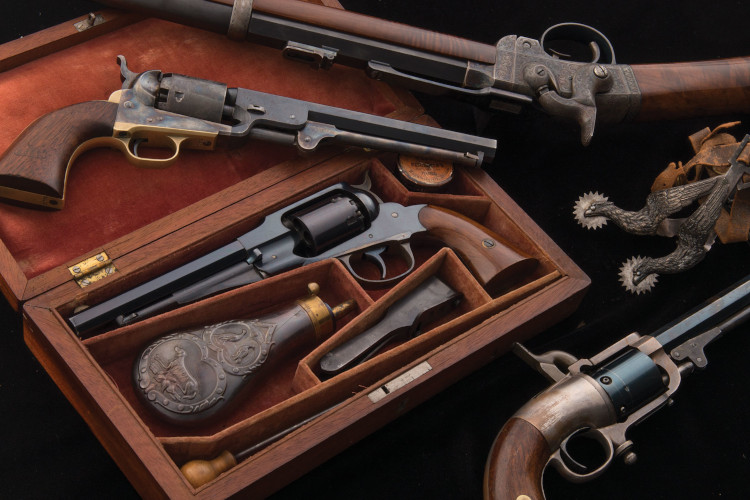This highly detailed color photograph, set against a stark black background, showcases an impressive collection of antique firearms and related paraphernalia. Dominating the composition is an exquisite wooden box, meticulously crafted with numerous compartments, each holding specific cleaning tools and supplies. Inside this open box lies an antique revolver, perfectly nestled within its designated space, exemplifying a well-preserved unit likely hailing from the 1800s. Atop the box's lid rests another revolver, casually positioned, adding to the historic ambiance of the display.

To the right of the wooden box, in the bottom right corner of the photograph, a different type of pistol is partially visible. Adding further intrigue, a long firearm, either a rifle or shotgun, stretches along the top border of the image, its length extending beyond the frame. Complementing this array of weaponry, a set of ornate silver spurs, adorned with eagle designs, can be seen at the periphery, contributing an additional layer of Old West authenticity and craftsmanship to the scene.